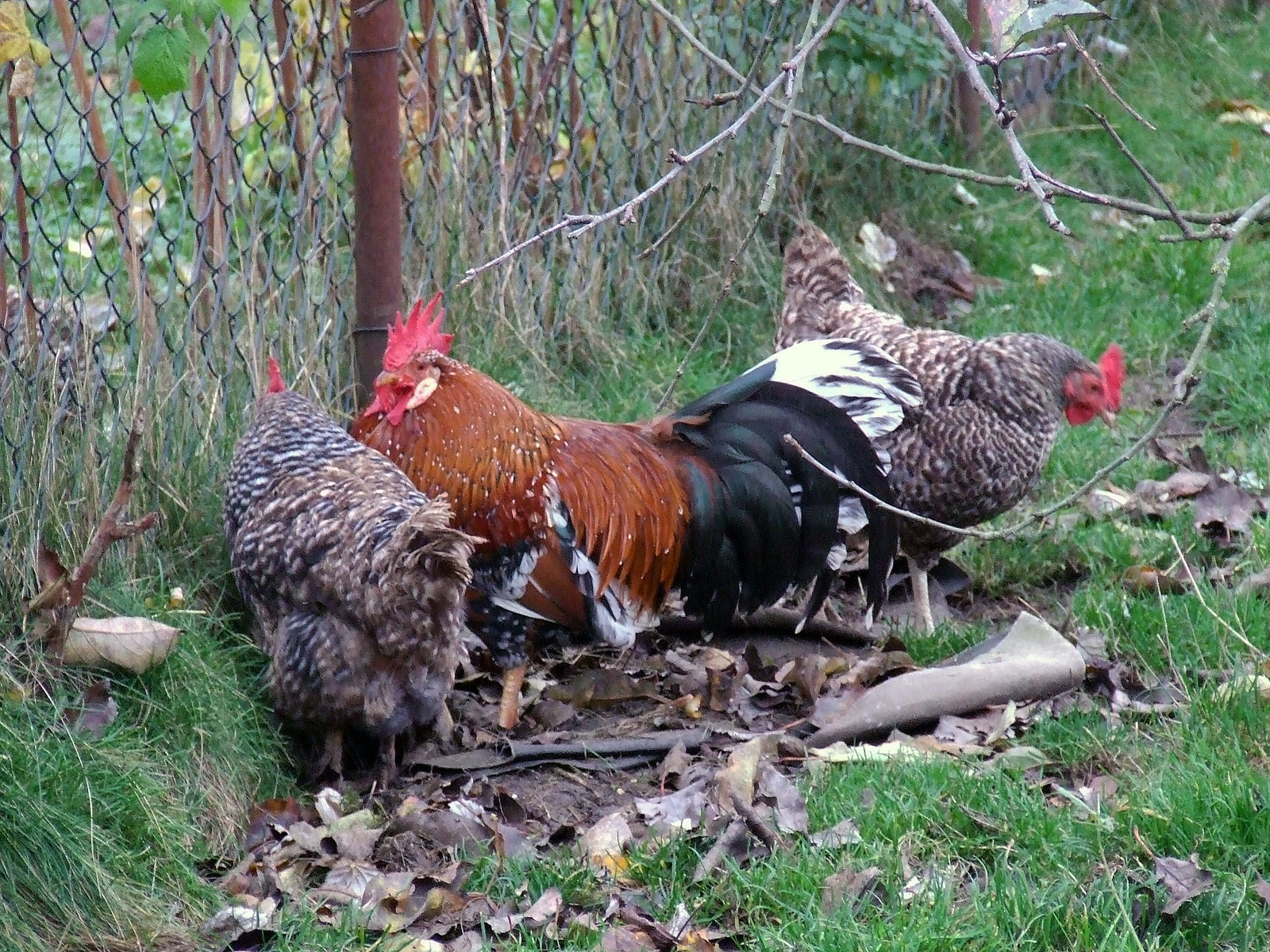In the image, three chickens are seen standing together in a lush, overgrown garden area with long grass and scattered leaves. Two of the chickens have speckled black, brown, and white feathers, while the one in the middle has striking reddish-brown feathers with a vibrant black and green tail that fans out. This middle bird, likely a rooster, boasts a prominent red crest and a red wattle underneath its beak, which is brown. The two speckled chickens also have red crests and facial features, with the one facing the camera showing a short yellow beak and the other being partly obscured. They all appear to be standing rather than feeding. In the background, there is a black chain link fence covered with plant life, intertwining sticks, and some leaves. The garden area is dense with greenery and some indistinguishable black and white objects scattered on the grass, possibly a tarp.